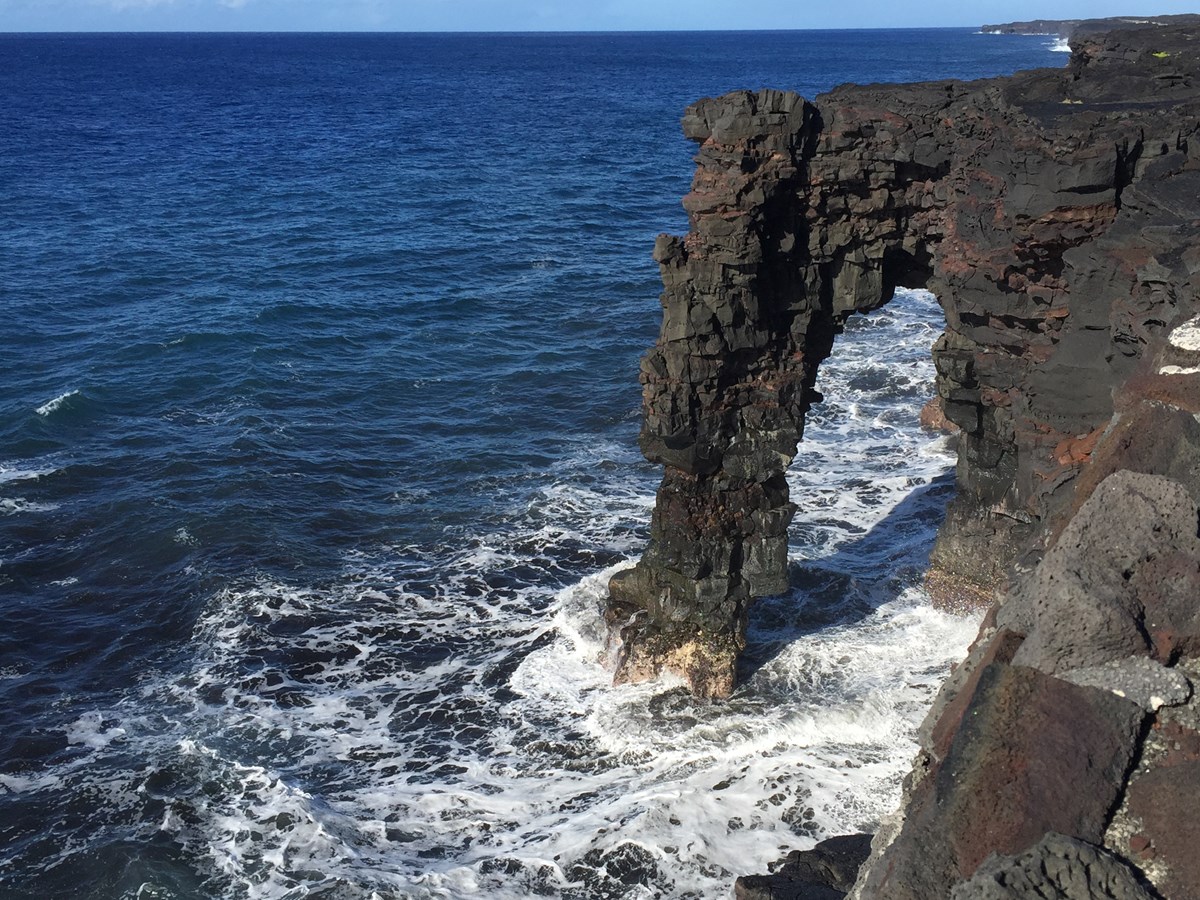This photograph captures a dramatic coastal scene where a striking natural rock formation meets the ocean. The image is taken from a high vantage point, looking down toward the water, which fills most of the frame with varying shades of blue, transitioning from dark to light. The ocean stretches out towards the horizon, a thin strip of blue sky visible at the top.

Dominating the upper right-hand corner is a prominent cliff composed of textured, rust, black, and gray rocks. Extending from this cliff is a naturally-formed stone archway, carved out by the relentless waves. Through this archway, the ocean can be glimpsed, creating a picturesque frame of blue water beyond. The rocks exhibit striking white streaks and spots, enhancing their rugged appearance.

Below the arch and towards the lower center of the image, waves crash into the rock formation, producing white foam and splash that contrasts with the azure water. The landscape is devoid of any vegetation or human-made structures, emphasizing the raw, untouched beauty of nature.